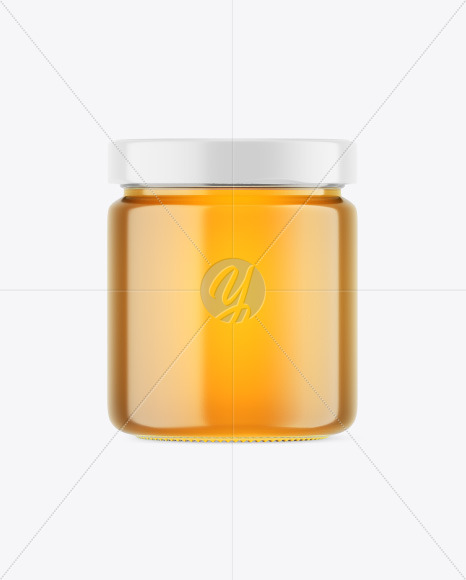The image features a square container made of clear glass, filled with a glowing, translucent yellow substance. The jar exhibits shades of brown particularly at the edges and vertically down the center. It is capped with a shiny, reflective silver lid. The background is plain white, which emphasizes the container. Intricately overlaid on the image are very light gray, intersecting diagonal lines forming a pattern, with an additional horizontal line crossing the diagonals at the center. At the focal point of this pattern is a circular gray logo centrally positioned on the container, featuring a cursive letter 'Y' in yellow. The entire setup gives a sense of the jar being slightly suspended in mid-air, due to the absence of any visible supporting surface.